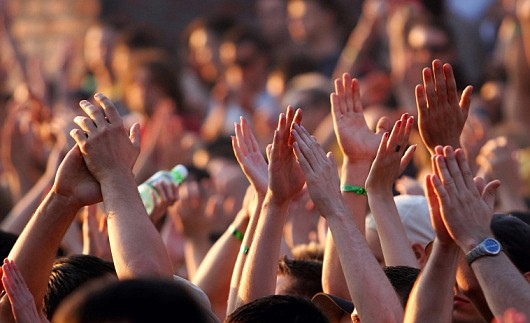This color photograph, in landscape orientation, captures a vibrant scene of a large crowd, likely at a concert or outdoor event, illuminated by natural sunlight. In the foreground, the image sharply focuses on multiple hands—approximately six to eight sets—raised high above heads, actively clapping in celebration. These hands, some adorned with watches and rings, dominate the middle section of the frame, displaying a sense of collective joy and unity. The individuals to whom these hands belong are visible from mid-forehead to the top of their heads. The background fades into a blur, showing a sea of other attendees, though their features and actions are less distinct. This photograph exemplifies photographic realism, capturing the essence of a jubilant moment within a large, diverse crowd.